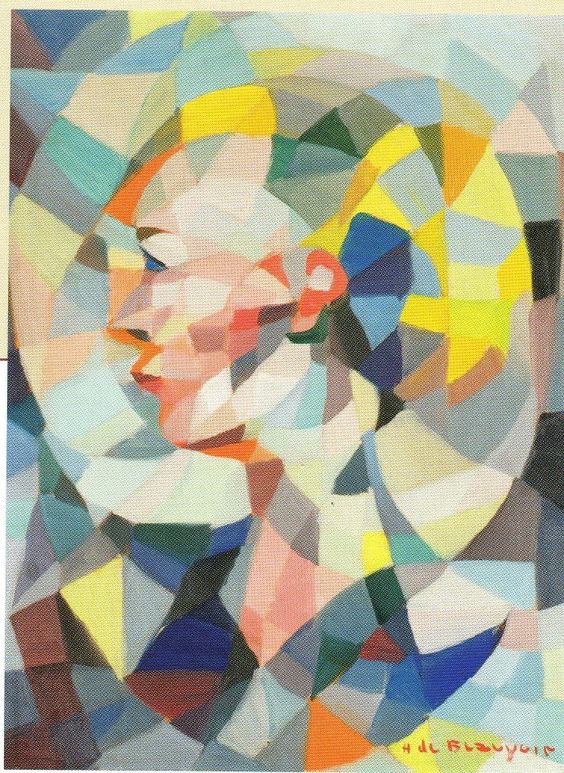This image is a vibrant and intricate abstract geometric painting on canvas. It captures the profile of a woman's face, oriented towards the left, with her striking blue eyes at the center of attention. Her face is composed of various geometric shapes—squares, triangles, and rectangles—in hues of white, yellows, oranges, reds, and blues. Her ear is highlighted in an orange tone, while her hair is rendered in yellowish shades, surrounded by a mosaic of concentric circles in diverse colors such as green, yellow, blue, and red. The overall composition features a swirling mosaic of solid colors and complex patterns, with the background blending dark greens, purples, and blues. The painting's texture reveals hints of the canvas beneath. Adding to the complexity, multiple halos emanate from her head, creating a dynamic and mesmerizing effect. The color palette is rich and varied, comprising golds, yellows, grays, blues, deep corals, oranges, maroons, and soft pinks. The portrait straddles the line between order and chaos, evoking the captivating and enigmatic nature of modern art.